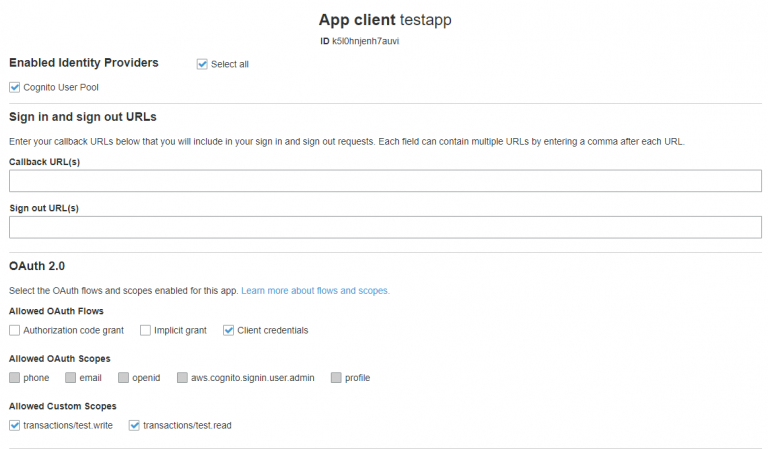A detailed and cleaned-up caption for the image could read:

---

The top center of the screen displays the title "App Client Test App". On the left side, there is a section titled "Enabled Identity Providers". Within this section, there is a selection box with a blue checkmark labeled "Select All". Below it, there is another selection box also with a blue checkmark labeled "Cognito User Pool".

A thin gray line separates this section from the next. Below the line, bold text reads "Sign In and Sign Out URLs". Immediately under this, there's an input field for entering "Callback URLs". The instructions specify: "Enter your callback URLs below. These will be included in your sign-in and sign-out requests. Each test can contain multiple URLs by entering a comma after each URL."

Further down, labeled in parentheses, are input blocks for "Callback URLs" and "Sign Out URLs", meant for data entry.

The next section is titled "OAuth 2.0". It has a description: "Select the OAuth flows and scopes enabled for this app." There is a link labeled in blue: "Learn more about flows and scopes." 

Below this, the "Allow OAuth Flows" section presents checkboxes for different flow options: "Authorization Code Grant", "Implicit Grant", and "Client Credentials", with "Client Credentials" being selected, indicated by a blue checkmark.

Next, the "Allowed OAuth Scopes" section lists several scopes: "Phone", "Email", "OpenID", "AWS Cognito Sign-In User", "Admin", and "Profile".

Lastly, there is an "Allowed Custom Scopes" section with selections checked for the scopes "transaction/tests.write" and "transaction/tests.read".

---